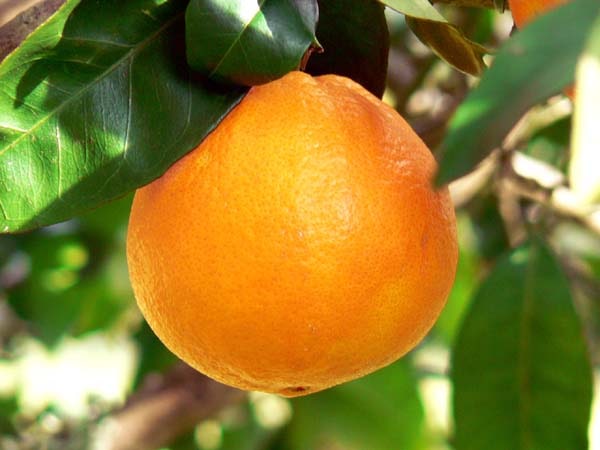The image features a vibrant, ripe orange still hanging from its branch, positioned slightly off-center towards the left of a close-up shot. Dominating the foreground, the orange's skin is smooth and a rich shade of orange, indicative of its freshness and readiness to be eaten. Surrounding the orange, in the upper left corner and partially framing it, are crisp green leaves that are in focus, adding to the natural aesthetics. The background is a blur of light and dark browns, greens, and occasional rays of sunlight filtering through, suggesting the setting is either in the wild or an orange grove. The overall scene is devoid of any text, focusing purely on the natural beauty of the orange and its surroundings.